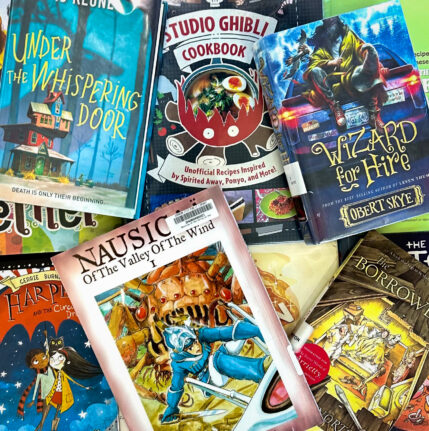In the image, we see a color photograph of a pile of books stacked horizontally, revealing their front covers. The collection predominantly features children's books and fantasy-themed titles, suggesting they could be from a library due to visible white spine labels and a barcode on one cover. Highlighting the fantasy theme, notable titles include "Nausicaä of the Valley of the Wind," "Wizard for Hire," and "Under the Whispering Door." Also partially visible in the stack is the "Studio Ghibli Cookbook," hinting at the diverse genres among the books. Although the titles and covers overlap, the vivid colors and intricate illustrations on each cover are distinguishable, making the display visually engaging.